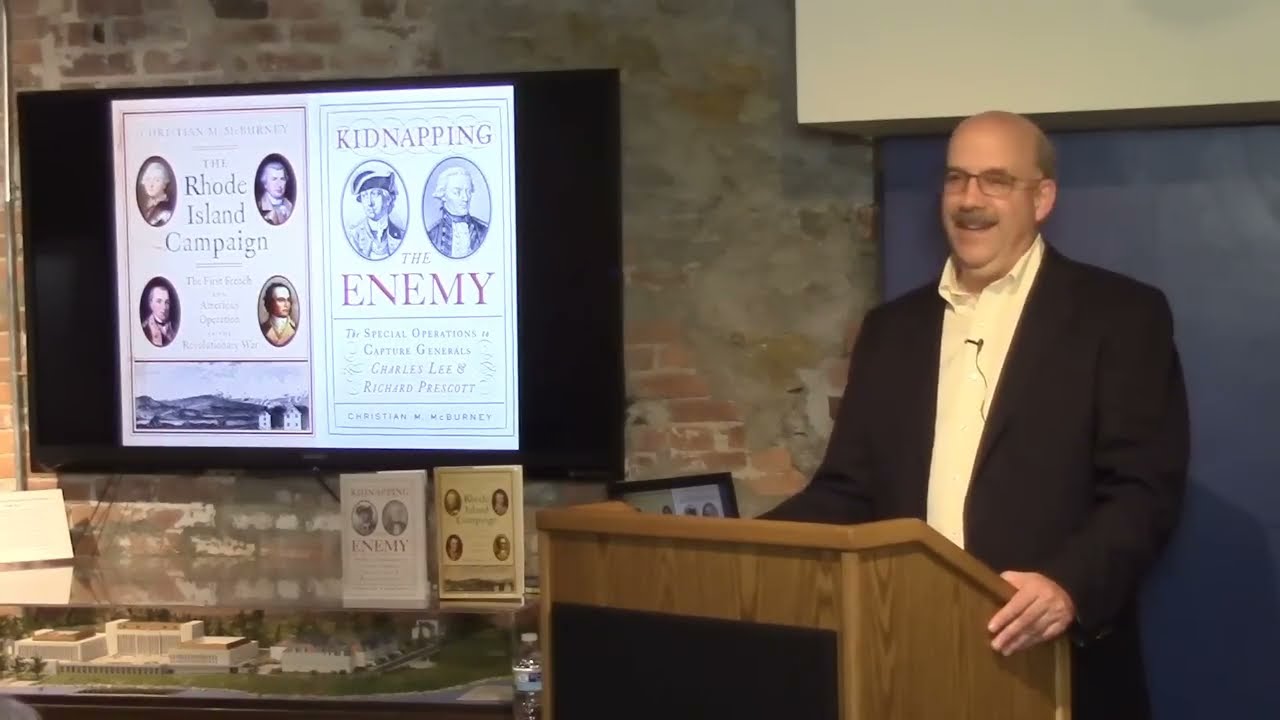The image depicts a middle-aged, bald, white man with salt-and-pepper hair and a gray mustache, standing at a wooden podium and delivering a lecture. He is wearing glasses, a dark blazer, and an off-white collared shirt. His hands are raised as he gestures animatedly while speaking. Behind him is a blue wall with a beige rectangular section above it. To his left, the background transitions to a red brick wall partially covered with gray plaster. Mounted on this brick wall is a black rectangular flat-screen TV displaying a vague black and white map. Below the TV, a table features a glass case containing a detailed model of a complex with white rectangular buildings, green grass, and small green trees. On top of the glass case, there are two books: a white one titled "Enemy" on the left and a beige one on the right.